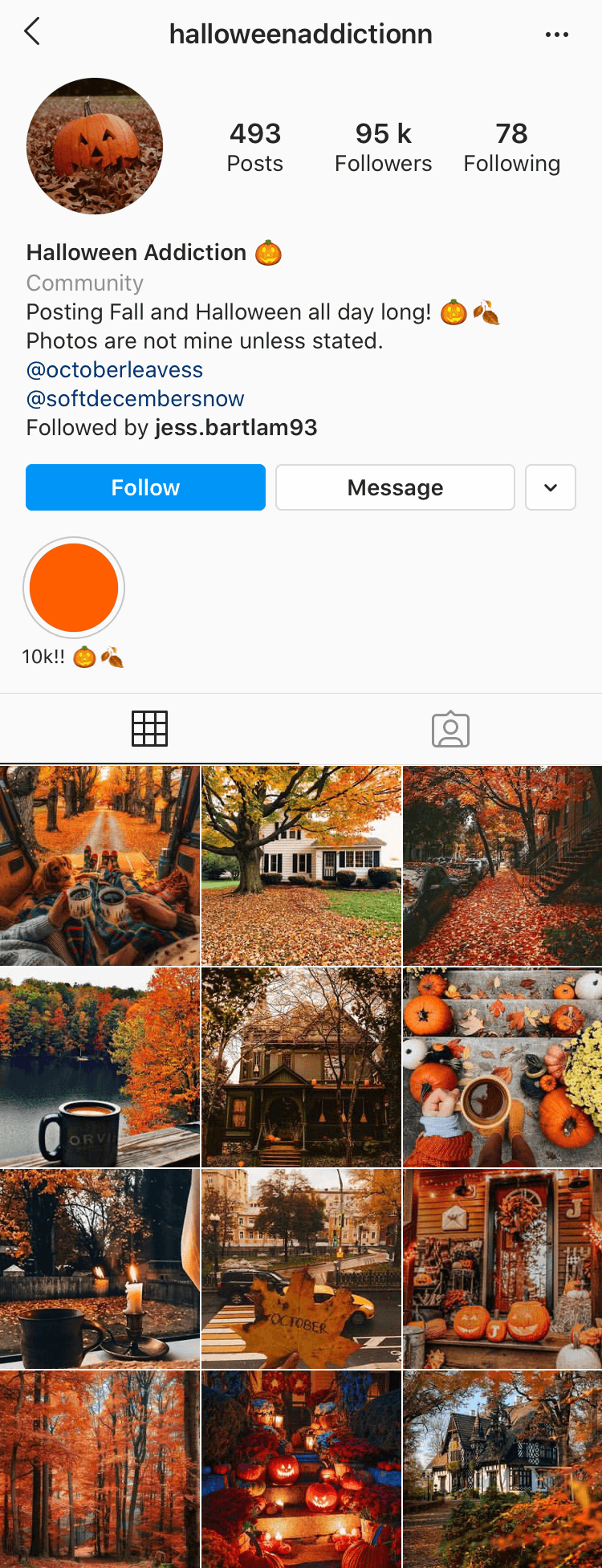**Halloween Addiction Instagram Profile Overview**

*Profile Name:* Halloween Addiction  
*Profile Picture:* Icon featuring a pumpkin and autumn leaves  
*User Activity:* 493 posts  
*Followers:* 95,000  
*Following:* 78

**Profile Description:**  
Halloween Addiction - Community dedicated to sharing everything about fall and Halloween. We post content full of autumnal vibes all day long! 🍂🎃

*Disclaimer:* Photos are not mine unless stated otherwise.  
*Additional Details:*
- Regularly features content from: @OctoberLeaves and @SoftDecemberSnow.
- Followed by notable user: jess.bartman93.
- Recent milestone: 10,000 followers, indicated by an orange circle on the profile.

**Gallery Summary:**
- *General Theme:* Autumn and Halloween.
- *Content Includes:* 
  - A series of 12 aesthetically pleasing autumn photographs.
  - Highlights include:
    - A picturesque scene of leaves scattered in front of a cozy house.
    - Rustic steps adorned with an array of pumpkins.
    - A serene walkway blanketed with colorful fallen leaves.
    - Breathtaking views of a tranquil lake surrounded by autumn foliage.
    - Vibrant city park scenes capturing the essence of fall.
    - Close-up shots of various pumpkins in different settings.

This Instagram page delivers a consistent feed filled with the warmth and beauty of the fall season, perfect for enthusiasts of autumn and Halloween.